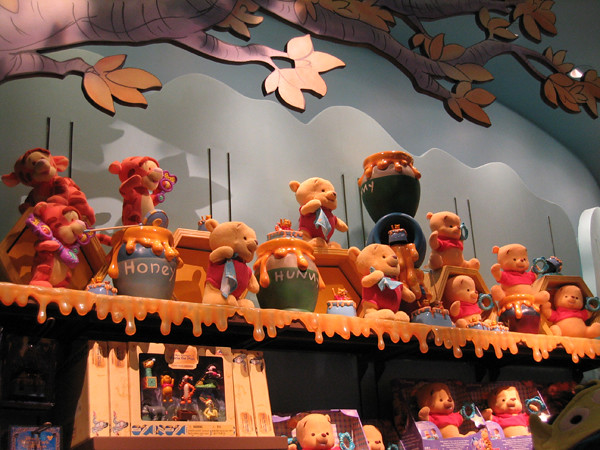The image captures a beautifully detailed and vibrant display inside what appears to be a Disney store, possibly located within Disneyland. This display features an array of Winnie the Pooh-themed items meticulously arranged on a shelf. The top shelf appears to be adorned with a tree bursting with orange leaves and a backdrop painted with blue skies and clouds, creating an enchanting woodland setting. Prominently featured are multiple stuffed Winnie the Pooh toys, each sporting his iconic red shirt and positioned in various playful poses. Interspersed among the Pooh toys are several jars of honey, some labeled humorously as "H-U-N-N-Y." To the left side of the display, there are also three Tigger stuffed animals adding to the charming scene. Below the main shelf, additional Winnie the Pooh toys are neatly packaged and displayed, ready for enthusiastic collectors. This delightful setup not only showcases a wide range of Pooh-themed collectibles but also immerses visitors in the magical, whimsical world of the beloved characters.